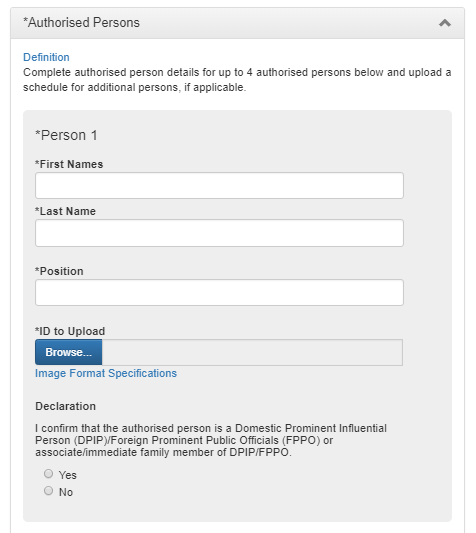The image depicts a detailed form layout for inputting information regarding authorized persons. The overall background is predominantly grey, providing a neutral backdrop. The fields intended for input are stark white, creating a clear contrast for easy readability.

The top of the form is labeled "Authorized Persons" with an asterisk indicating mandatory fields. Below, there is an instruction to complete the details for up to four authorized persons, with an option to update the schedule for additional entries if necessary.

The form starts with "Person 1" and includes fields for:
- First Name(s)
- Last Name(s)
- Position ID

There is an option to upload an image, with a blue button labeled "Browse" to facilitate selecting an image file.

Further down, there is a "Declaration" section, where the user is required to confirm whether the authorized person is a domestic prominent influential person (DPIP) or a foreign prominent public official (FPPO), or if they are an associated immediate family member of a DPIP/FPPO. There are two radio buttons—one for "Yes" and one for "No"—positioned vertically, allowing the user to make the appropriate selection. 

Throughout the form, the colors used are grey, black, white, and blue, which highlight different sections and buttons effectively.